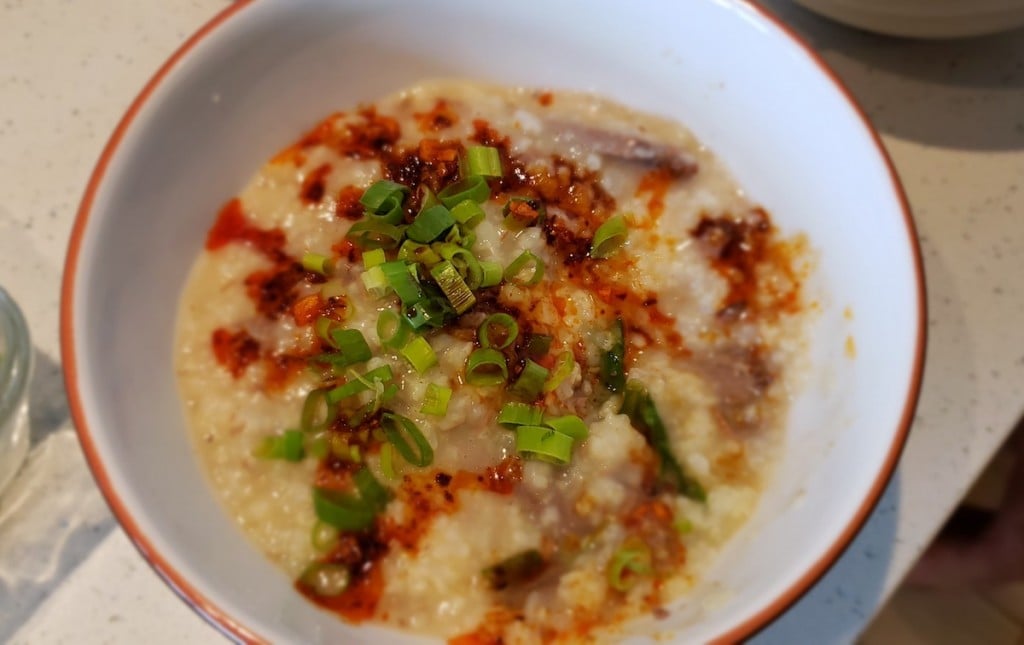This photograph captures a detailed close-up of a food bowl placed on a speckled white and gray surface. The bowl features a white interior and a red rim, complementing its colorful contents. Inside the bowl, there appears to be a semi-liquid dish resembling khichdi or a creamy, grain-like mixture such as couscous, with off-white, red, and orange hues. The dish is garnished with chopped green vegetables, likely cilantro or green onions, and is generously topped with a red sauce or hot sauce. 

The white and black speckled countertop provides a contrasting backdrop to the vibrant bowl and its contents. Within the composition, the edge of a clear glass is visible on the left side, and the partial view of another white bowl is discernible in the upper right corner. Shadows from these items cast softly onto the countertop, adding depth to the scene. The overall image is a rich and detailed portrayal of a flavorful dish presented in a simple yet colorful bowl, set against a lightly speckled surface with hints of surrounding utensils.